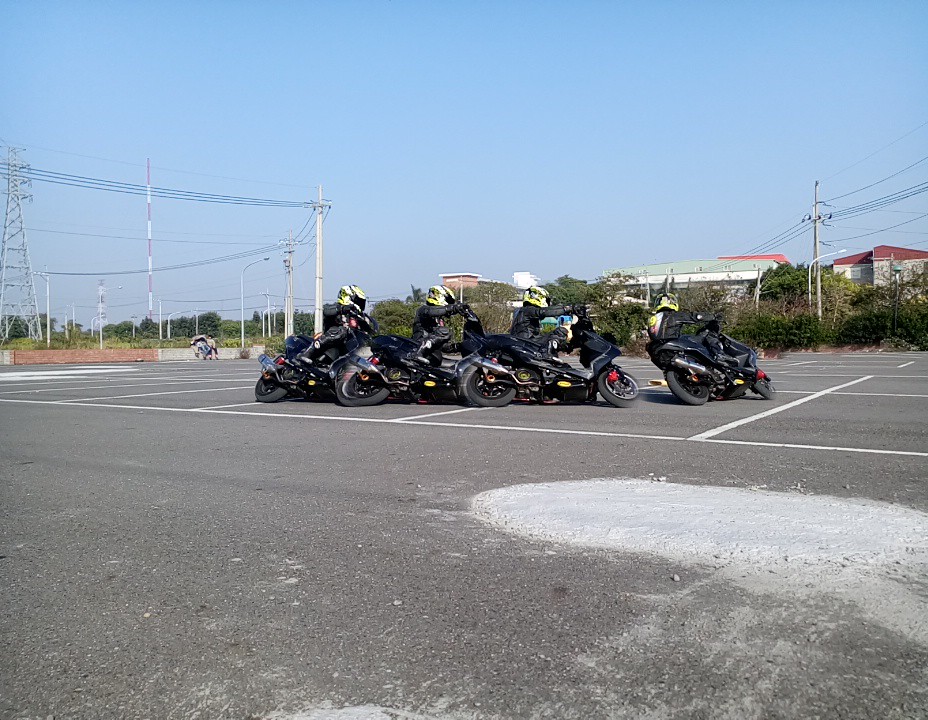In this detailed outdoor image, a group of four motorcyclists is prominently featured on a stretch of black asphalt that appears to be a temporarily repurposed parking lot or road intersection. The riders are executing a tight circular formation, leaning left as if navigating a curve. Each motorcyclist rides an identical dark navy blue bike with black wheels and wears a matching black leather jacket. They sport yellow helmets, adorned with black markings for added visibility. In the foreground, particularly in the bottom right corner, there is a conspicuous large, smeared spot of a light gray or white powdery substance—possibly recently poured cement.

In the background, a line of trees and bushes extends across the width of the scene, beyond which rooftops of various colors—dark red, light red, light green, and white—are visible. Further still, numerous power lines stretch across the horizon, accompanied by a distinctive radio tower standing tall in the far upper left corner. The image not only captures the dynamic activity of the motorcyclists but also provides a rich tableau of the surrounding landscape, emphasizing both the immediate action and the distant scenery.